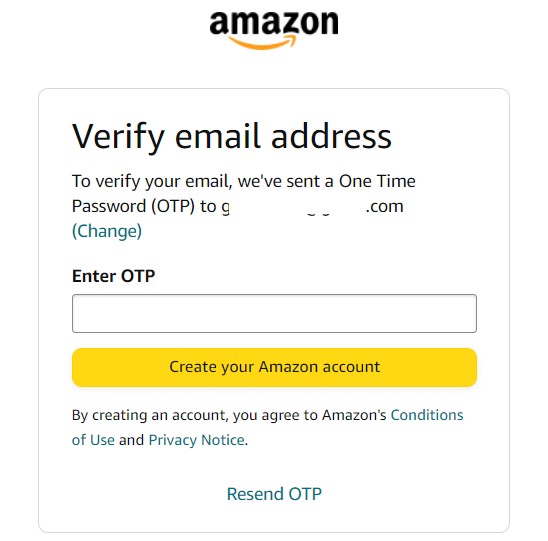At the top of the image, the word "Amazon" is displayed in black text, accompanied by the iconic small yellow arrow that originates from the letter 'A' and curves to point underneath the letter 'Z'. Immediately below, within a square, the text reads "Verify Email Address". 

To proceed with the email verification, there are instructions stating: "To verify your email, we've sent a one-time password (OTP) to [email protected]." Below this message, a line in parentheses says "change", highlighted in blue, allowing the user to modify the email address if necessary.

Next, the image prompts with the text "Enter OTP", fully capitalized, under which an empty input field is provided for the user to enter the one-time password. 

Further down, there is a prominent yellow oval button that contains the text "Create your Amazon account". 

At the bottom of the image, in black text, a statement reads: "By creating an account, you agree to Amazon's", followed by "Conditions of Use" and "Privacy Notice" in blue text, indicating hyperlinks. Approximately three inches lower, also in blue text, is the option "Resend OTP" for users who may not have received the initial email.